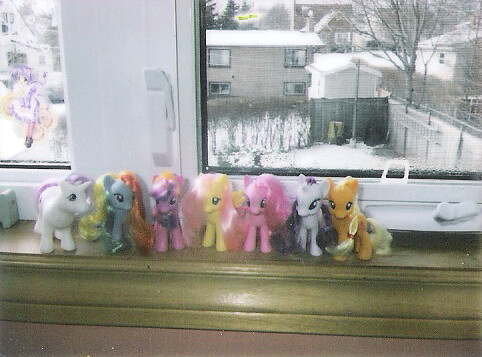On a wooden windowsill sits a vibrant collection of eight My Little Pony figurines, perfectly arranged and facing the camera. Each pony, made of colorful rubber, has distinct characteristics: a white pony with purple hair, an orange pony with a white mane and tail, a yellow pony with pink hair, a blue pony with rainbow hair, and several pink ponies with various hair colors, including one with pink and another with purple. Their bright, almond-shaped black eyes add to their expressive appearance. Behind them, through white-framed windows, a wintry scene unfolds with snow blanketing the ground and rooftops of the houses and buildings outside. The morning light illuminates the snow, adding a serene backdrop to this charming display. A tree is visible on the far right, contributing to the picturesque winter landscape.